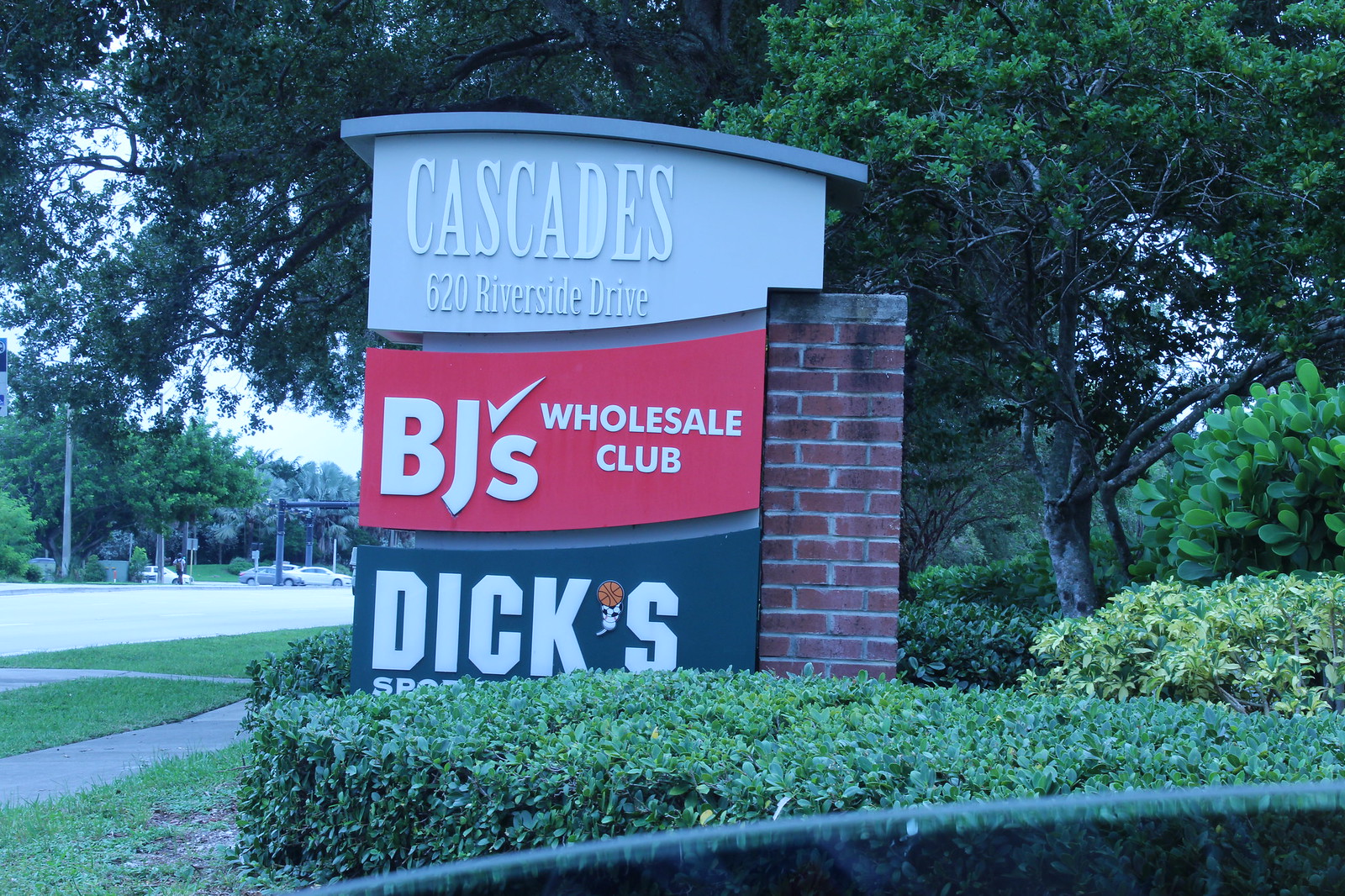The image shows a high-class sign located outside the Cascades Shopping Center at 620 Riverside Drive. The sign, supported by a brick column on the right, features three main panels: the top panel in white text reads "Cascades, 620 Riverside Drive;" the middle panel in a red section displays "BJ's Wholesale Club" with a checkmark serving as the apostrophe; and the bottom panel shows "Dick's Sporting Goods," although the "Sporting Goods" portion is partially obscured by well-manicured shrubs. Additional neatly trimmed shrubs also surround the sign and extend behind it. The scene, captured through the rolled-down window of a car, features a clear, sunny day, with numerous trees and bushes in the background. On the left side of the image, you can see a sidewalk running parallel to the road, which has cars stopped at an intersection in the distance. Overall, the picture portrays a well-maintained and visually appealing entrance to the shopping center amidst lush greenery.